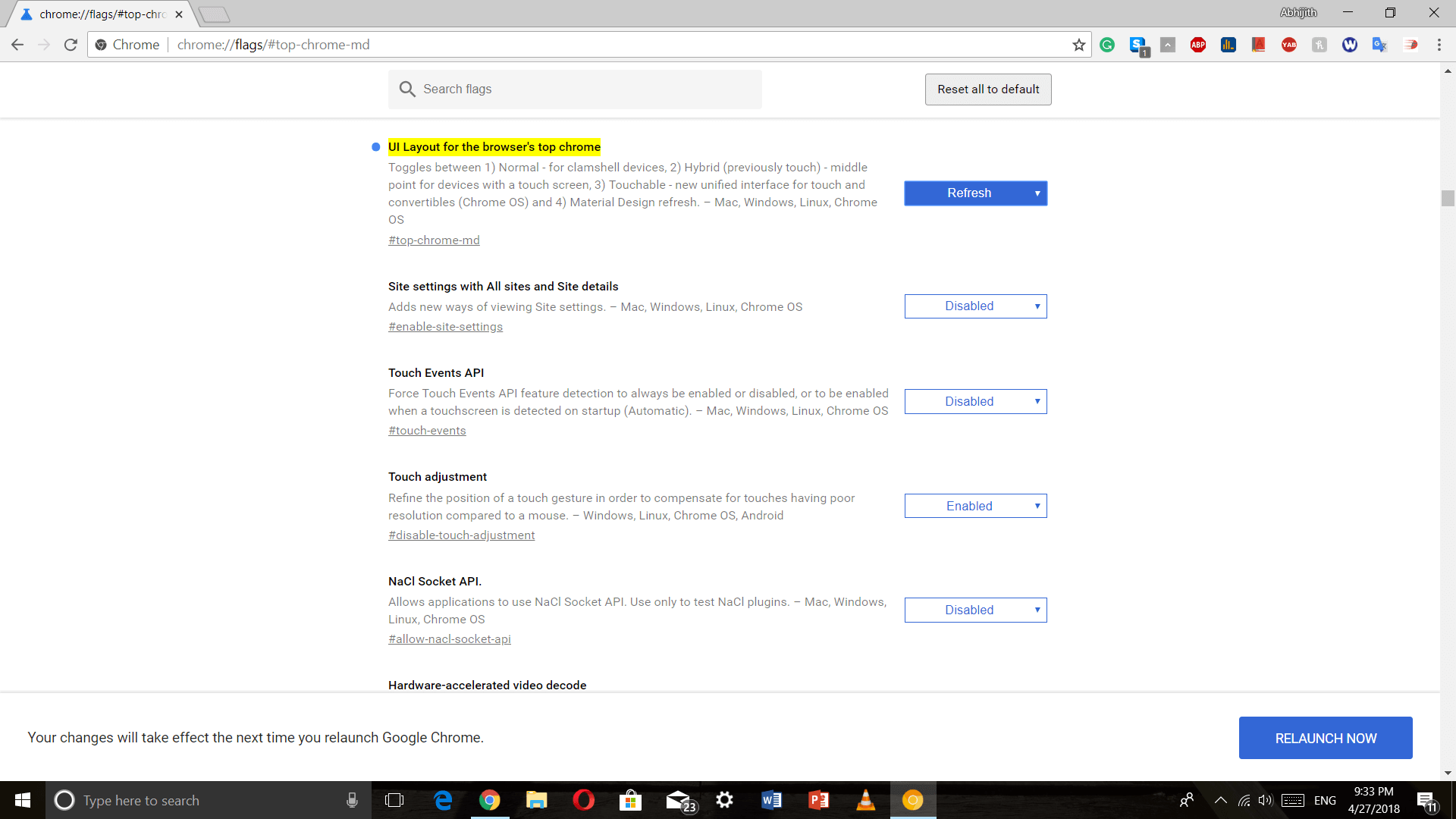This image displays a web browser interface, specifically a Google Chrome tab. The tab seems to have a blue profile icon on the left and possibly displays "Chrome" or a related term that starts with the letter 'C'. The browser's address bar shows a URL that includes "chrome://flags/", indicative of the Chrome Flags settings page. Adjacent to the URL is a star icon for bookmarking, followed by several miscellaneous icons.

Beneath the address bar is a light gray navigation banner, and below that, a white banner appears. Centrally located within this white banner is a search bar with a faint magnifying glass icon on the left and the placeholder text "Search flags" inside. To the right, outside the search bar, is a button labeled "Reset all to default."

Highlighted in yellow within the main content area is an entry titled "UI Layout for the browser's top Chrome," accompanied by a blue dot to its left. Below this title is a descriptive paragraph. To the right of this entry is a blue refresh button with a drop-down arrow.

Further down, the page lists various subtitles and settings options, including "See sheet settings with all states and site details." Additional settings such as "Touch adjustment," "Touch events API," and "Selected API" are also noted, each with its respective state shown in a dropdown menu allowing for enabling or disabling the features.